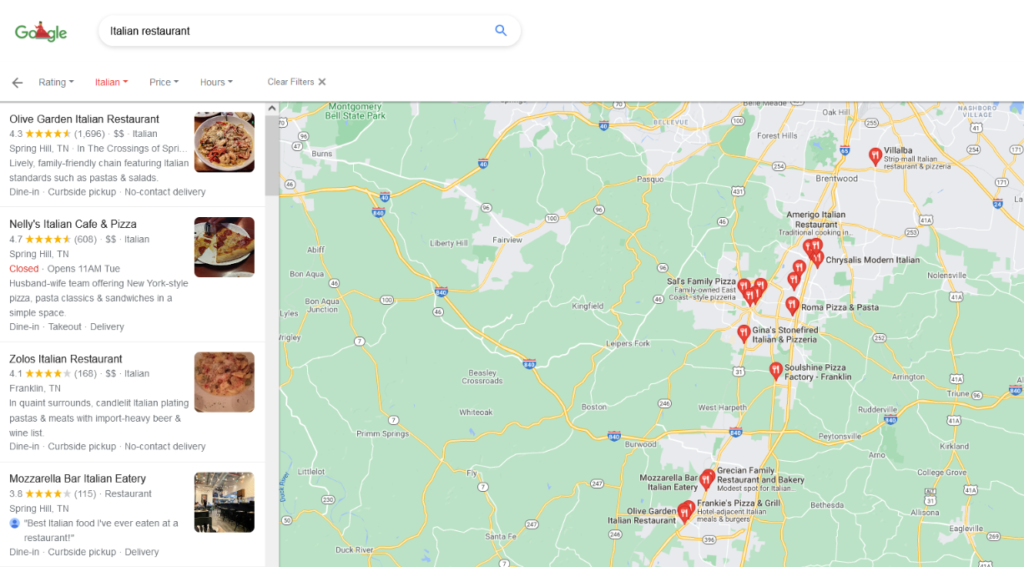The image depicts a Google search results page for "Italian restaurant." At the top, there is a menu bar featuring rating filters, an Italian cuisine drop-down menu, price ranges, operating hours, and a clear filter button to reset the search parameters. Below this section, on the left side, a series of individual restaurant listings are displayed. Each listing includes the restaurant's name, a small square image (either of a meal or the restaurant itself), and additional details in their descriptions. Notable restaurants in the results include Olive Garden Italian Restaurant, Nelly's Italian Cafe and Pizza, Zulu's Italian Restaurant, and Mazzarello Bar Italian Eatery. Although the image is cropped and the scroll bar indicates there are many more listings, only these four are immediately visible. To the right, there is a larger image encompassing multiple restaurants, with an estimated 15 to 20 different eateries shown within the screen’s visible area.